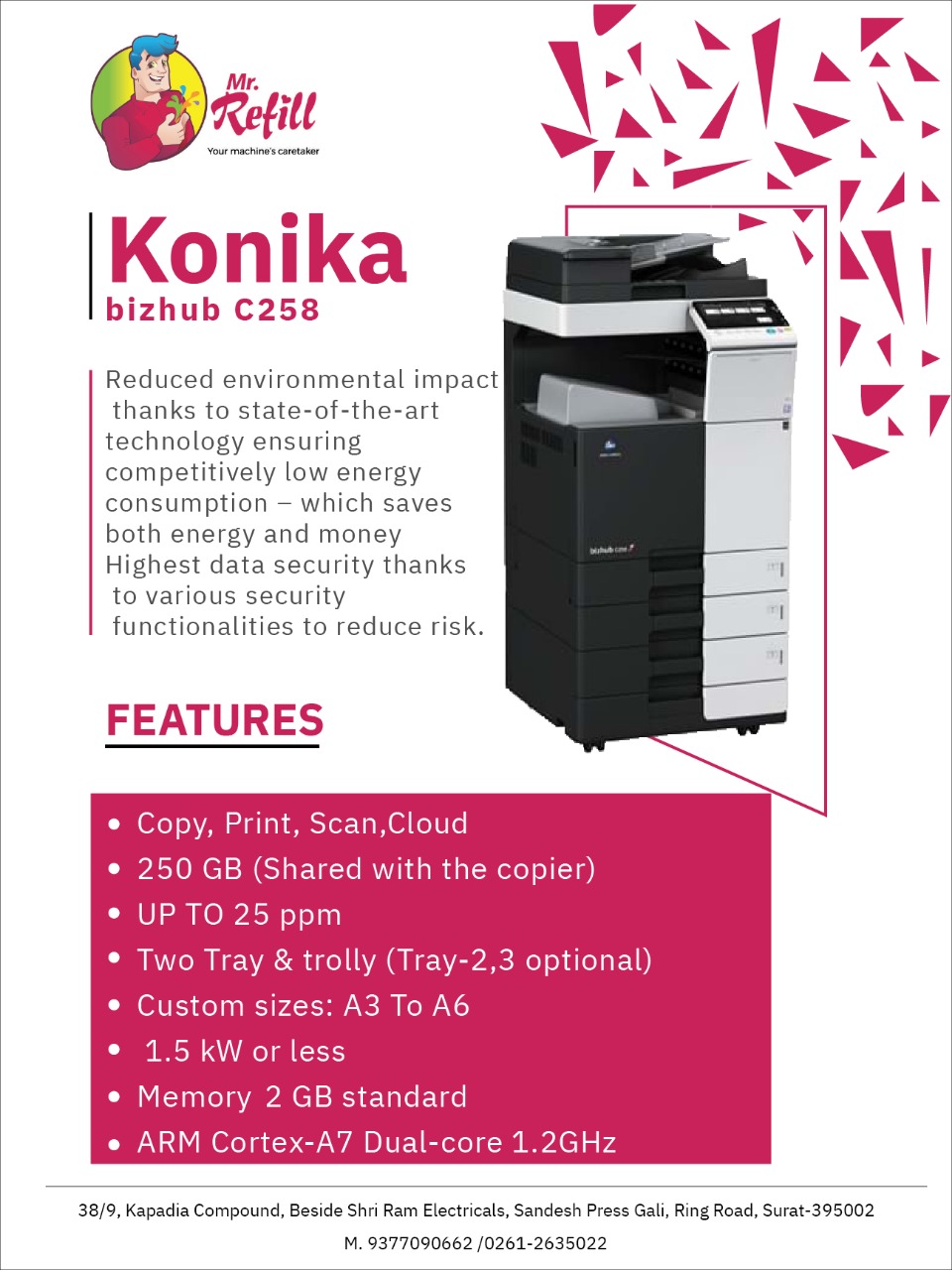This advertisement poster features the Konica BizHub C258 copier, prominently displayed to the right as a tall, black and silver, bulky office printer with wheels. To the top left is the logo of Mr. Refill, illustrated as a cartoon man with blue hair, wearing a red shirt, and the tagline "Your machine's caretaker" beneath it. The text highlights the product name, Konica BizHub C258, and emphasizes its eco-friendly technology that reduces environmental impact through low energy consumption, saving both energy and money. It also stresses the highest data security features to minimize risks. Key features listed in a red text box include copy, print, scan, cloud capabilities, 250 gigabytes of shared storage, a print speed of up to 25 pages per minute, two trays with an optional third tray and trolley, custom paper sizes ranging from A3 to A6, a power consumption of 1.5 kilowatts or less, standard memory of 2 gigabytes, and an ARM Cortex-A7 dual-core 1.2 GHz processor. The bottom of the poster includes contact details for obtaining the product from the company.